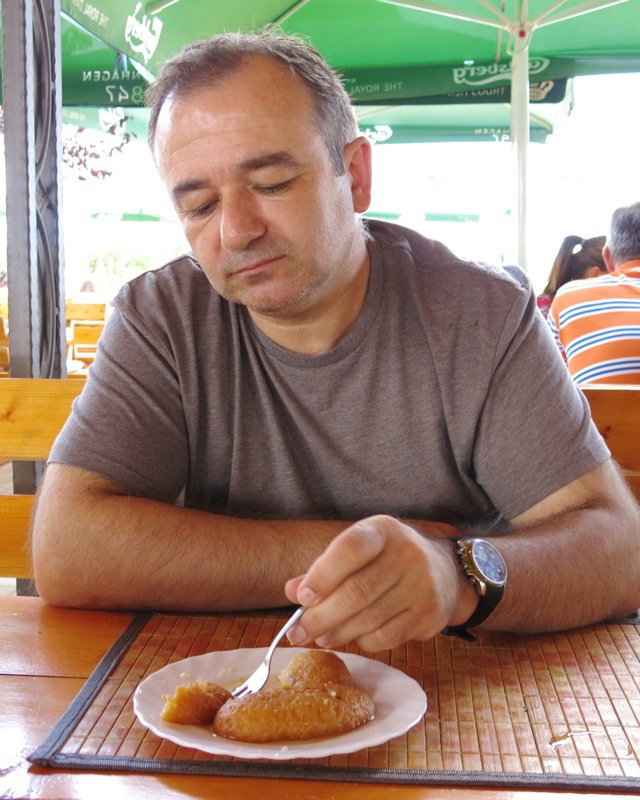In this detailed photograph, a middle-aged man, possibly in his 50s, is enjoying a meal at a restaurant's outdoor patio. He has short, thinning brown hair with hints of gray and wears a grayish-brown shirt. The man has tan skin and hairy arms, and sports a stylish black watch with a gold face. Seated on a bench-style seat with wooden paneled back and table, the man appears to be in mid-action, using a fork in his left hand to cut into a pastry-style dessert that is served on a white plate over a bamboo placemat with a gray border. The dessert looks cakey with a lumpy texture and is swimming in a sauce or syrup.

In the background, there are green canopies with indistinct white writing, possibly pertaining to the restaurant’s branding. Nearby, white umbrella supports stand tall, confirming it’s a shaded patio setting. Additionally, a table with two other patrons is visible; one man is in an orange, blue, and white striped shirt, and another person, a woman, is wearing a red top and has her hair in a ponytail. With a half-smile and nearly closed eyes, the man gives off a relaxed vibe as he indulges in his dessert, likely captured by the person sitting across from him.